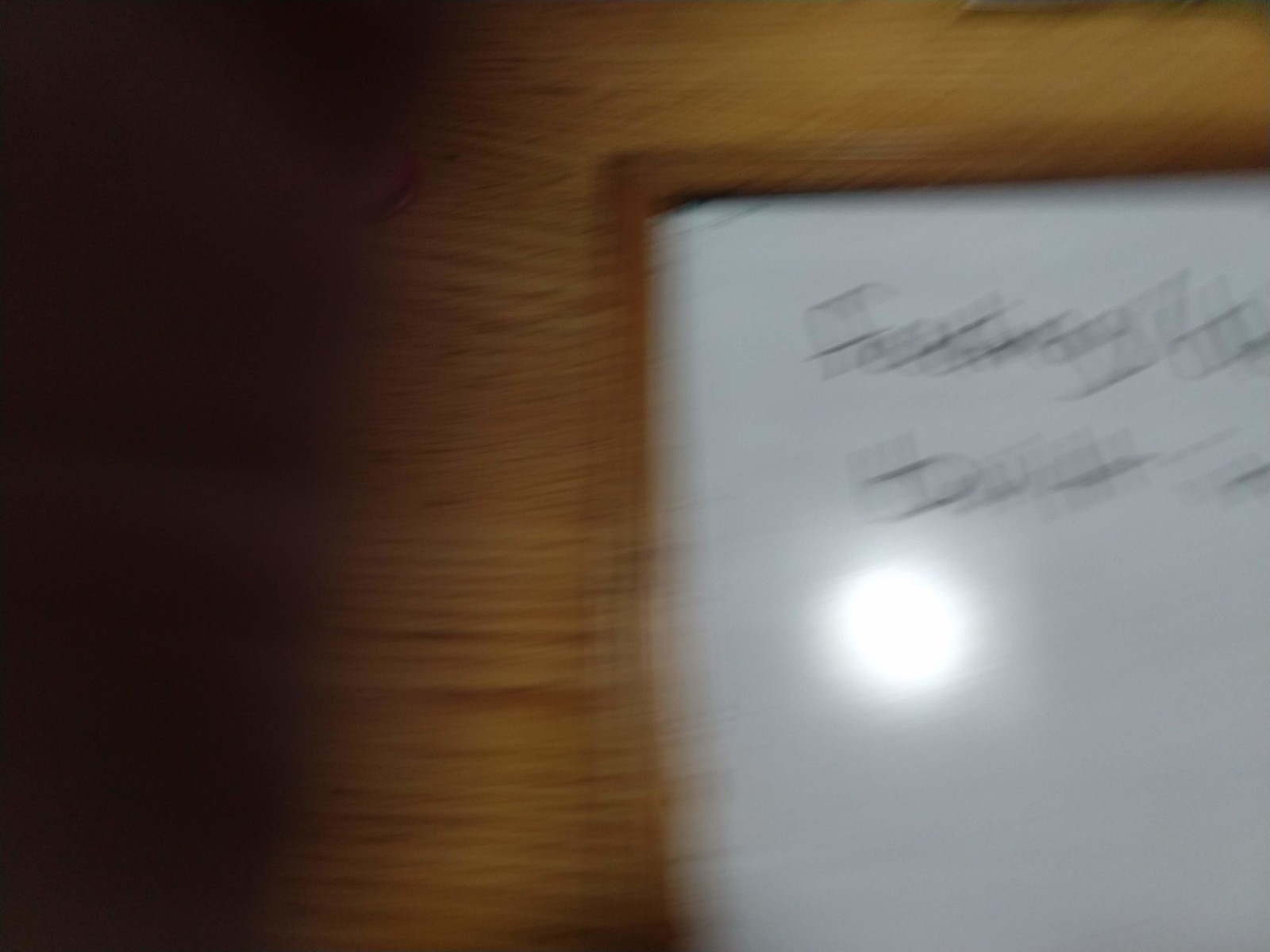The image captures a very blurry photograph of what appears to be a whiteboard, positioned on a wood grain tabletop that is likely artificial. The grains of the wood are oriented horizontally. The whiteboard extends from the right side of the image and covers about half of the photo, starting roughly a quarter of the way down and stretching in a straight line toward the left. There is a bright, circular light reflected on its glossy surface, indicating it's not made of paper. Despite the blur, two lines of writing in black—presumably from a dry erase marker—are faintly visible, though illegible. The left side of the image is dominated by a large, indistinct dark shadow, further obscuring details.